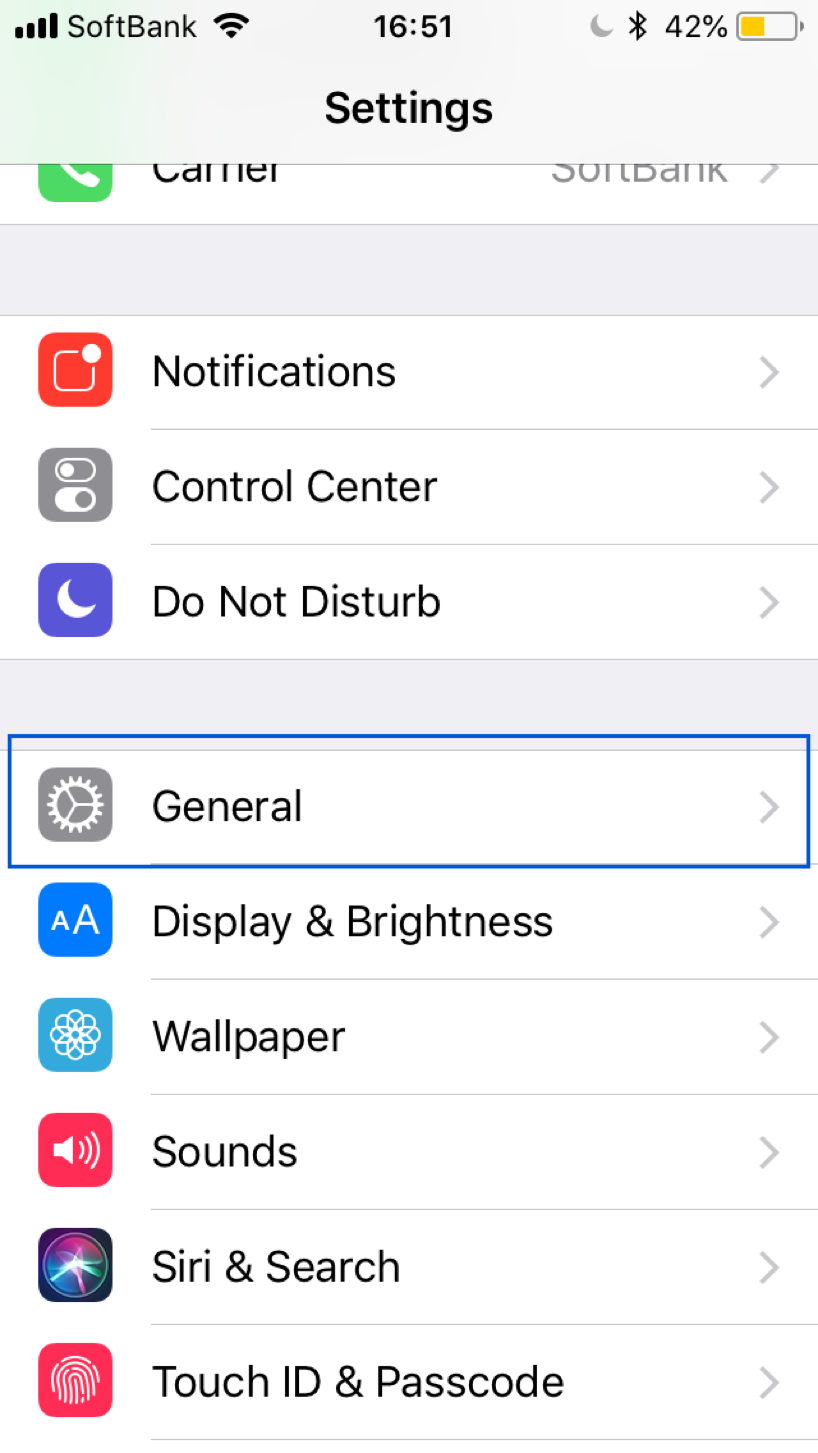The image, captured on an iPhone with SoftBank as the service provider, displays the Settings screen at 16:51, with the battery life showing at 42%. The phone is set to "Do Not Disturb" mode, indicated by the purple moon icon. The device itself is gold in color. 

The Settings menu is organized in a column of icons and text against a white background. At the top, "Notifications" is represented with a red icon, followed by "Control Center" shown with a gray icon. Next is the "Do Not Disturb" option marked by a purple moon. "General" settings are indicated by a gear icon. "Display & Brightness" features two capital A's in a blue icon, while "Wallpaper" is marked by a teal icon with a flower image. "Sounds" is represented by a red icon with a megaphone emitting lines, suggesting sound. Following that is "Siri," which has a multi-colored icon in pink, green, and blue with a white burst of light in the center. Lastly, the "Touch ID & Passcode" option is depicted with a pinkish thumbprint icon.

Overall, the detailed arrangement of the icons and clear depiction of each setting option make for a comprehensive overview of the iPhone’s Settings screen.